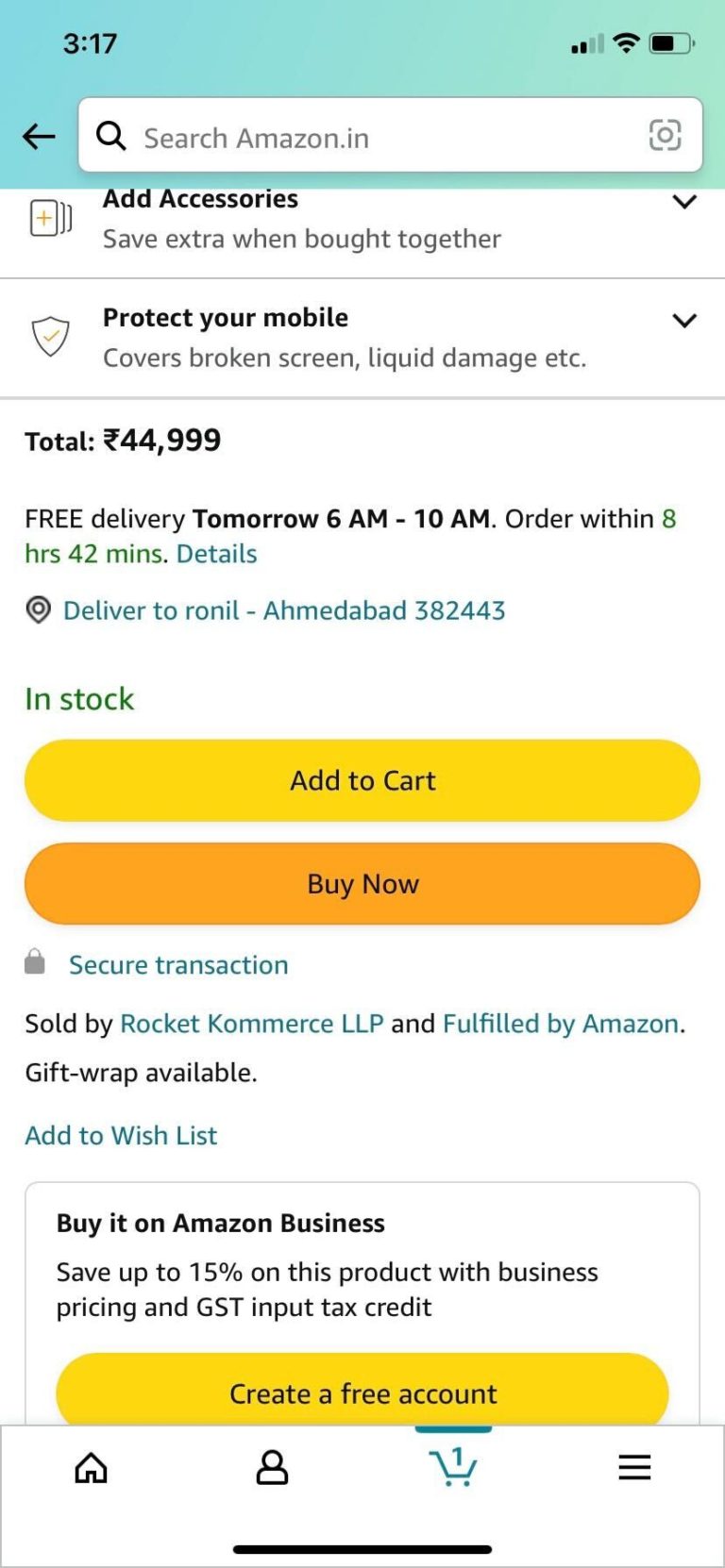The image displays a smartphone screen with the Amazon India app open. At the top of the screen, set on an aqua-blue background, the time is marked as 3:17 PM. To the right, indicators for network signal strength, Wi-Fi status, and battery life (approximately 60% charged) are visible.

Beneath this, a navigation bar features a black left-pointing arrow on the left and a white search bar containing a magnifying glass icon with the text "Search Amazon.in" in grey. Adjacent to the search bar, there is a photo icon.

The main section of the screen highlights product purchasing options. Visible is a segment indicating "Add accessories" coupled with a drop-down menu. Below, another drop-down pertains to "Protect your mobile." The total cost for the selected items is displayed as Rs. 4,999, suggesting the currency is Indian Rupees.

Underneath the cost, it mentions free delivery available for the following day between 6 AM and 10 AM. The product is in stock and is set to be delivered to Ronil in Ahmedabad, with the postal code 382443. 

Options to "Add to Cart" or "Buy Now," marked as a secure transaction, are prominently displayed. At the very bottom of the screen, navigation options allow the user to access "Home," "My Account," "Cart," and another section not clearly specified in the description.